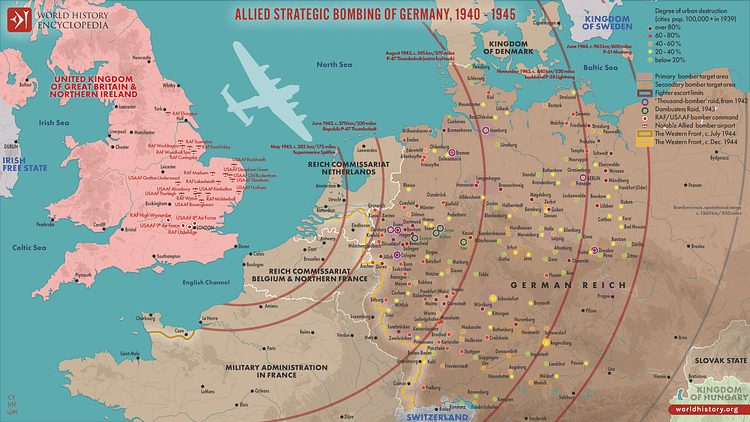This detailed illustration is a horizontally oriented map depicting the Allied strategic bombing of Germany from 1940 to 1945. At the center, prominent red text highlights the caption, "Allied Strategic Bombing of Germany 1940 to 1945." Germany, shaded in brown, features numerous cities marked with yellow circles and black text. The central region of the map is labeled "German Reich" in black. Across the German territories, red arc-like shapes indicate the bombings. A light blue, detailed image of a World War II plane is shown flying from the United Kingdom, labeled in pink, towards Germany. In front of the plane, "North Sea" is inscribed in blue. The top left corner of the map features a red square logo, accompanied by the black text "World History Encyclopedia." The map itself uses a color gradient to denote degrees of urban destruction and population, ranging from dark red to green, representing over 80% to below 20%. Complementary geographical regions like the United Kingdom of Great Britain and Northern Ireland, Kingdom of Denmark, Reich Commissariat, Belgium, Northern France, and the military administration in France are also highlighted.